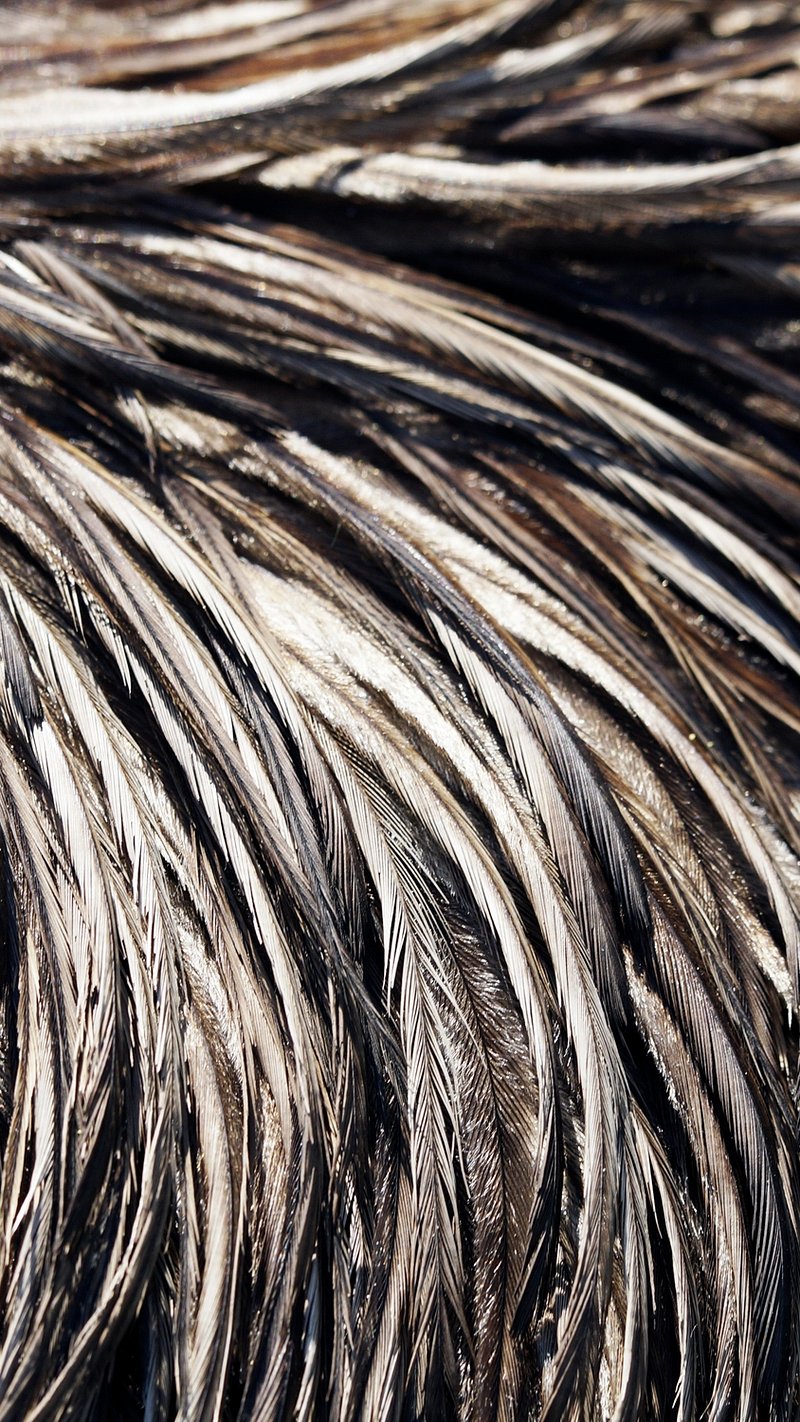The image is a detailed close-up of bird feathers, possibly from a wild bird like a hawk. The photograph prominently displays hundreds of feathers in varying hues of black, brown, white, and some beige. The feathers are layered, with many pointing downward and a few pointing upward at the top of the image. Some appear damp, giving them a golden sheen under the light, and they arc gracefully from the upper left to the bottom of the rectangular frame. The intricate arrangement and different layers create a rich tapestry of color and texture, illuminated in such a way that adds depth and dimension to the feathers. No other features are visible in the image, focusing solely on the complex beauty of the feathers.